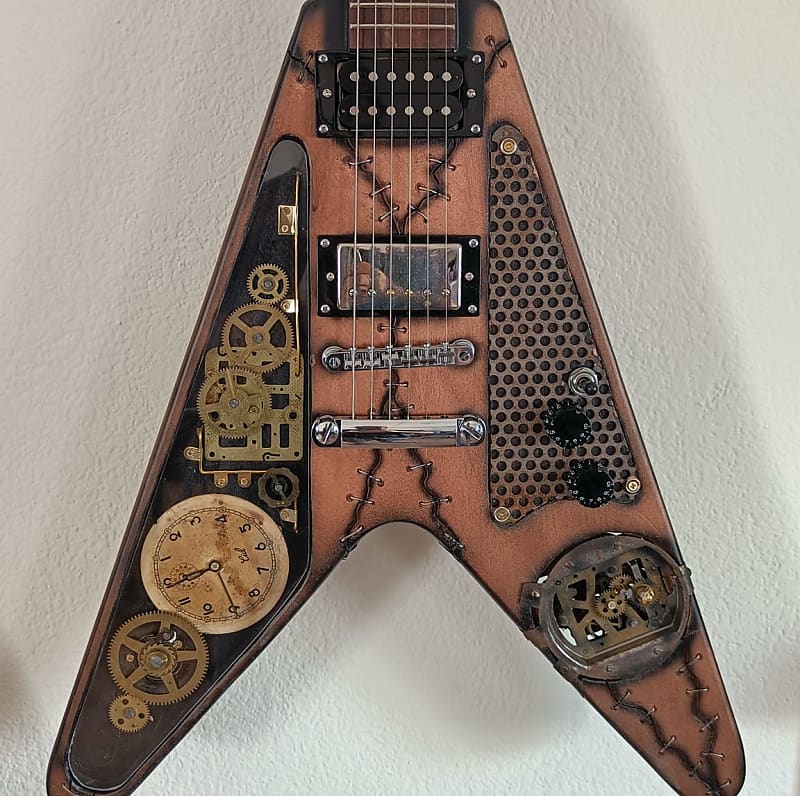The image depicts a steampunk-styled electric guitar adorned with intricate mechanical designs. The left side features a prominent antique clock face at the center, surrounded by multiple interlocking gold gears. These gears and clock components add an elaborate, vintage dimension to the guitar’s aesthetic. On the bottom right, there are smaller gears encased in a metal frame, and above them is a grill, secured by rivets at three corners, enhancing the mechanical theme. The top portion of the guitar, below the strings, displays a row of small dots reminiscent of capacitor tops, suggesting an electrical component influence. The guitar strings are anchored at the bottom with visible screws. The body of the guitar itself appears to be dark wood with black lines and a design that mimics stitched-together, patchwork triangles, accentuated by metal 'staples' running along the seams, evoking a Frankenstein-like appearance. The right side of the guitar also features staple-like marks and seams, giving the instrument a rugged, patched-up look. The combination of these elements creates a cohesive and highly detailed steampunk aesthetic.